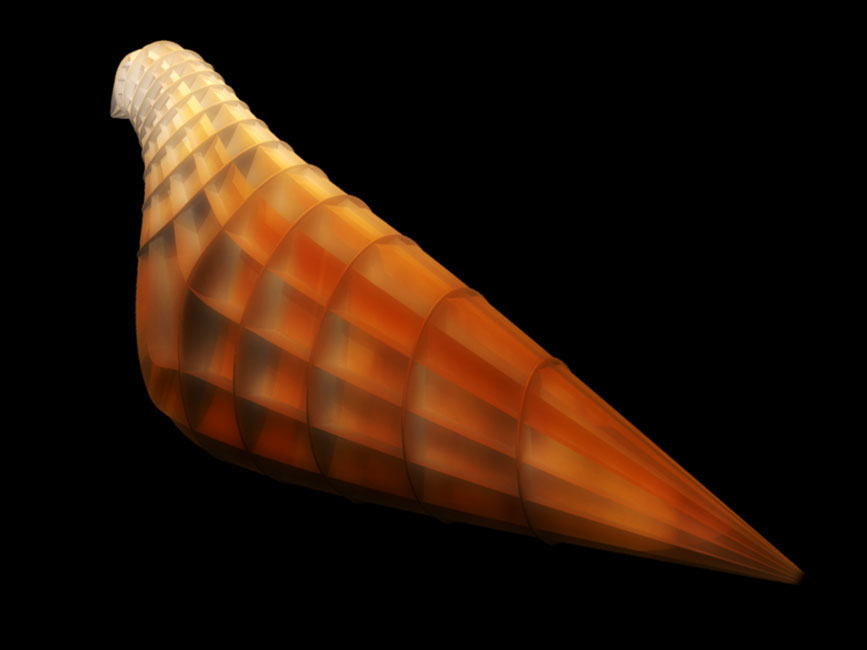The image depicts a detailed decorative sculpture resembling a bird, set against a completely black background. The sculpture features a head that mimics a bird with a distinct beak, starting in white and transitioning through a gradient of yellow, light orange, and medium orange before reaching the body. The body of the bird showcases a harmonious blend of dark orange, red, and yellow tones, arranged in a segmented, honeycombed pattern. The tail, located at the bottom right, is composed of vibrant reds and yellows. The entire sculpture, with its oblong shape and upward curling form, gives the impression of an intricately colored shell with an ombre effect from white at the head to darker hues at the tail.